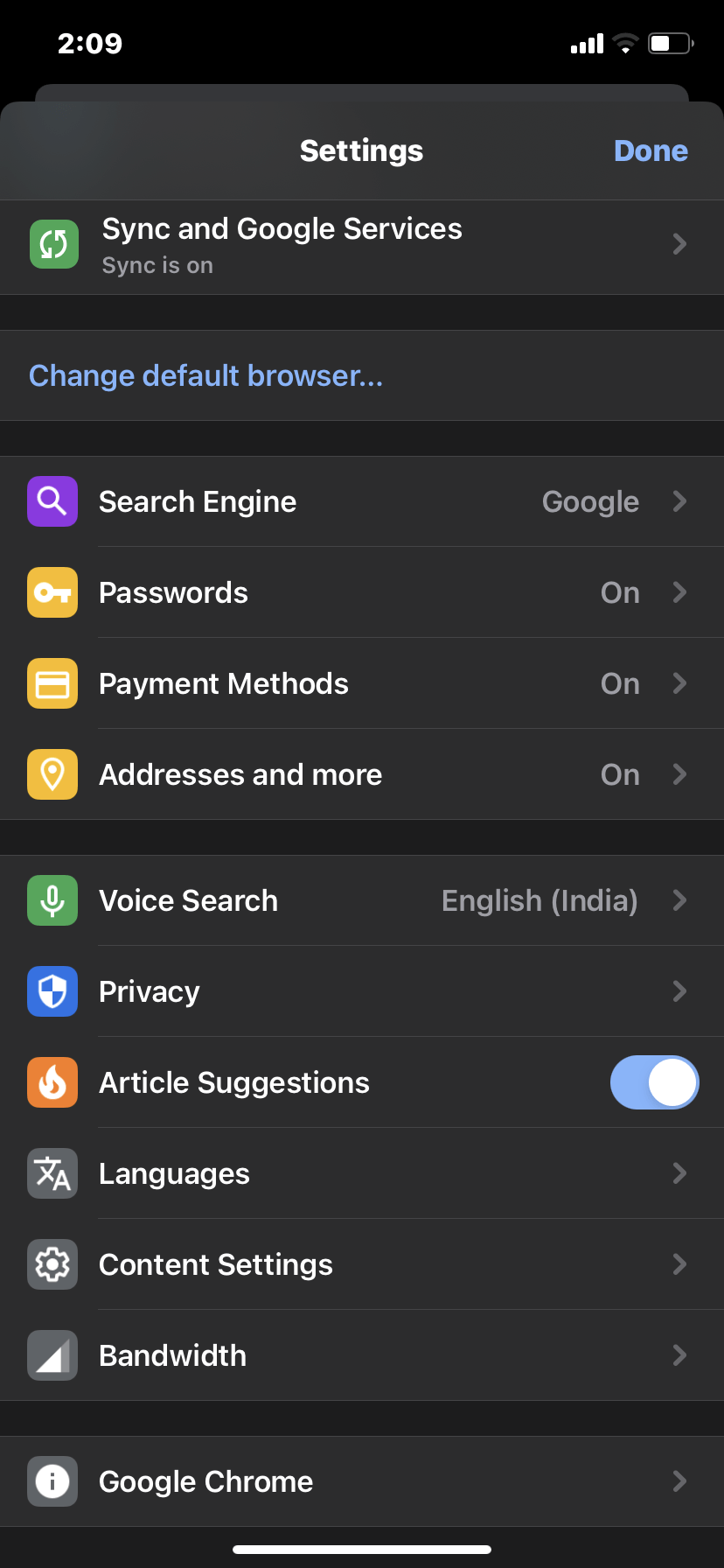Screenshot of Android Settings in Dark Mode 

The screenshot displays the Android settings interface in dark mode, featuring a black background. Key elements include:

- The upper left corner shows white text '2:09'.
- The upper right corner indicates cell phone signal strength, a small white dot, and a half-full battery icon.

In the central section:
- The word 'Settings' is displayed prominently.
- To the right, 'Done' is highlighted in blue.

Settings Details:
- 'Sync and Google services' is displayed prominently with 'Sync is on' written in gray underneath.
- Below, a blue link labeled 'Change default browser' is visible.
- Further options listed include 'Search engines', 'Passwords' (in white), 'Payment methods' (in white), with their corresponding status 'on' in gray.
- Under the 'Search engines' heading, 'Google' is noted in gray, representing the current search engine selection.

Additional Settings:
- 'Voice search' is listed in white with 'English (India)' in gray.
- 'Privacy' settings and 'Article suggestions' (on) are present along with a blue toggle line and a white circle.
- Options for 'Languages', 'Content settings', 'Bandwidth' are listed toward the bottom.
- The very bottom displays 'Google Chrome' with a white dividing line.

This detailed visualization highlights the structured layout and interface elements of the Android settings menu in dark mode.